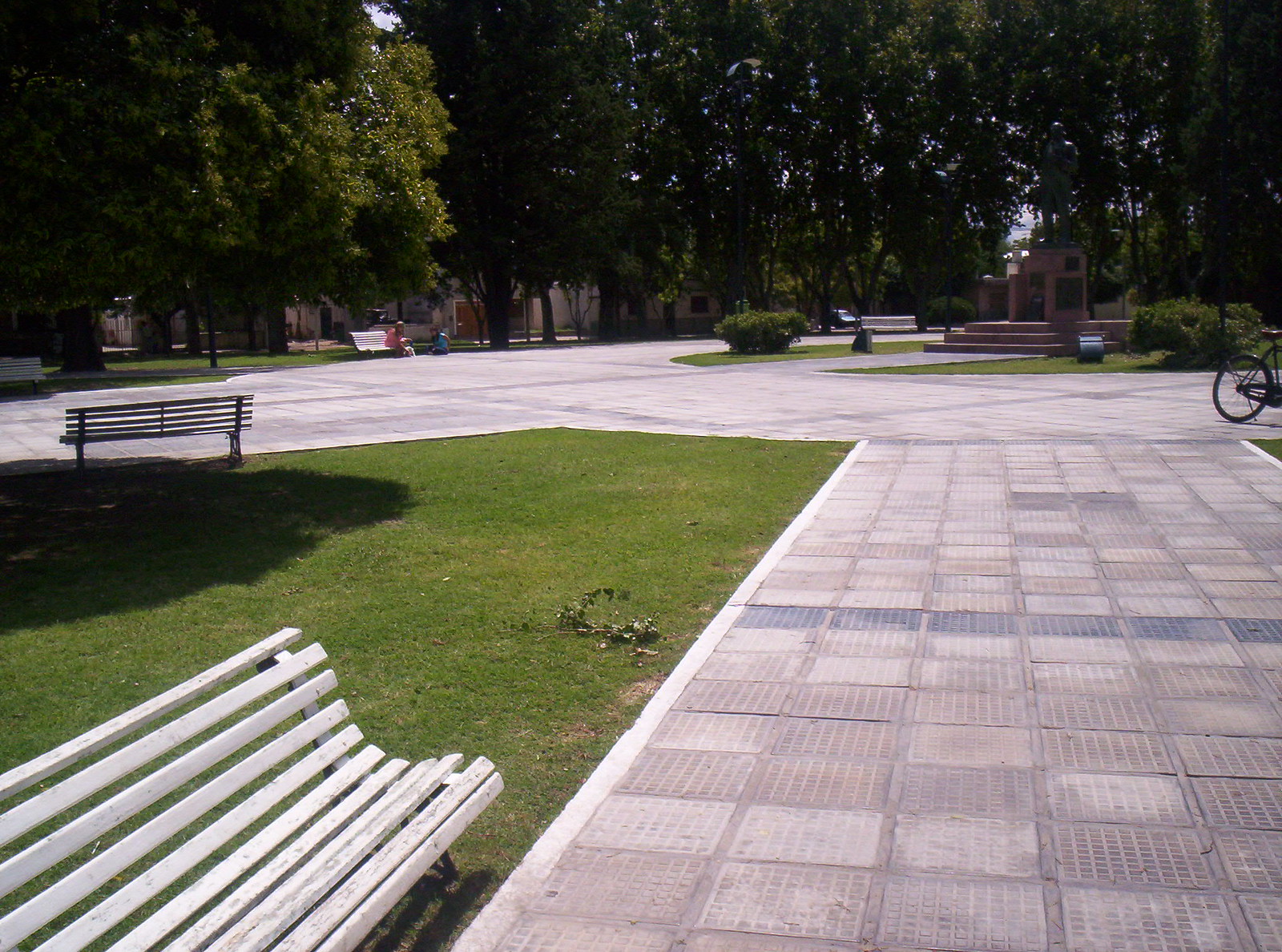In this large square picture taken outside, we see a park setting that resembles a courtyard with a blend of natural and constructed elements. On the left-hand side, green grass stretches out, and in the lower left-hand corner, a light gray wooden bench is partially visible. Beyond this grassy area, there is another bench facing away, positioned towards the left side of the image.

The entire middle and right side of the picture is dominated by a decorative walkway composed of square blocks in shades of light gray, light brown, and the occasional blue. Around this central path, the sidewalk leads up to a small memorial area with a few steps, perhaps featuring a plaque.

In the middle right of the image, you can spot the back wheel and seat of a bicycle. The background is densely lined with tall trees, presenting dark green leaves that appear almost black due to the shade. Despite the foliage, glimpses of the sky peek through, although it's unclear if it's sunny or cloudy. 

There are also a few people in the scene: one person sits on a bench beneath the trees, conversing with another person seated on the ground. The environment is further enriched with additional benches; one is shaded under a tree in the grass, and another is noted for its positioning close to the foreground on the left. In the far background, some buildings are partially obscured by the dense tree line, adding layers and depth to this quiet park moment.